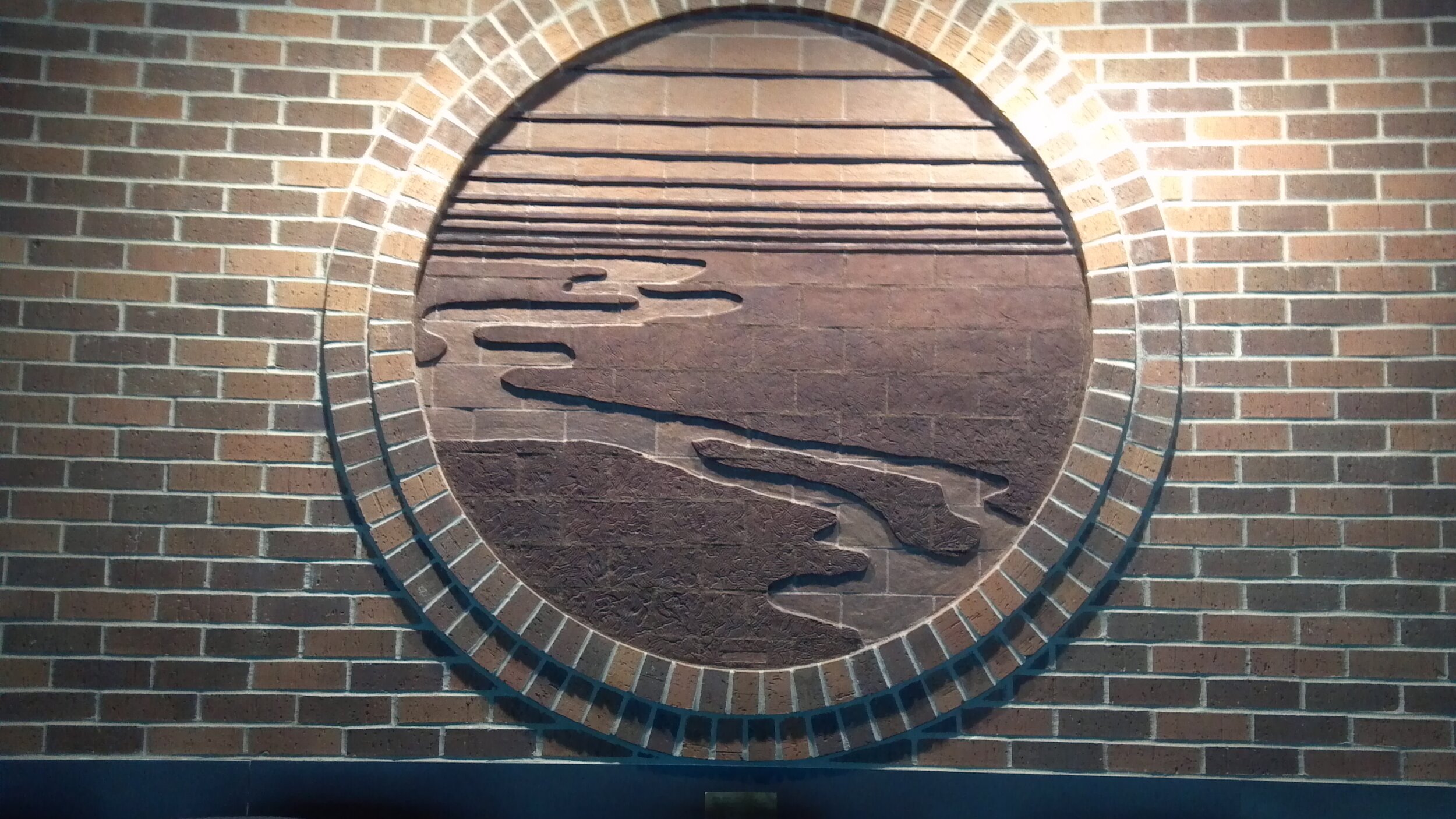The image depicts a brick wall comprised of various shades of bricks, ranging from tan to medium brown and darker chocolate brown, all separated by white grout. Dominating the center of the wall, there is a distinct circular frame made of two rows of bricks. Within this circular brick frame, there is an intricate design resembling a scene with wetlands, featuring dark land areas and lighter gray water sections. The bricks in the background of this design evoke a sky-like appearance. The lighting is notably poor, suggesting either an indoor setting with inadequate illumination or a nighttime scene with a flash. No people or animals are present, placing full focus on the uniquely designed brick wall, suggesting there's more significance to the wall beyond its ordinary appearance.